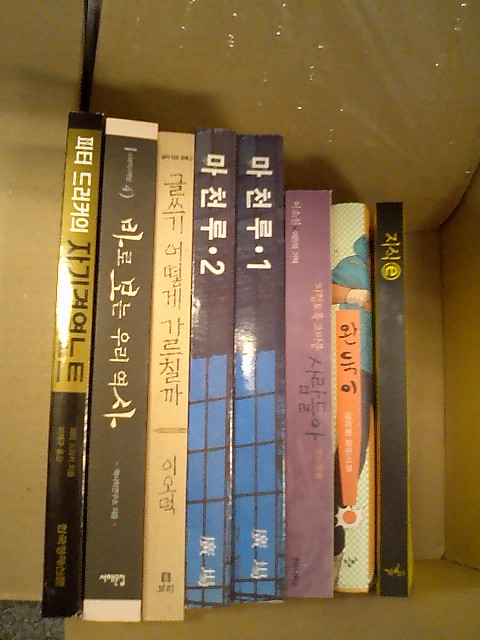The image depicts eight paperback books standing vertically inside a beige to gray cardboard box. These books feature Asian scripts, likely Chinese or Japanese, on their spines. Arranged by descending size from left to right, they vary widely in color and style.

- The tallest book on the far left has a black spine with gold Asian characters at the top, transitioning into a mustard color with additional black and white text.
- Next is a black and brown book with white text at the top and bottom.
- The third book is entirely cream-colored with black writing.
- The fourth and fifth books are a matching set, marked as volume one and two. They feature black spines with blue rectangle designs at the bottom and white text along the top, separated by dots and numbers one and two.
- Following the set is a shorter, maroon book with some black aspects.
- Next, there's a white book with an orange label and part of an illustration showing a person's arm or shoulder.
- The smallest book on the far right has a black spine with small gold Asian characters.

The overall impression is of a collection of distinctly different books, visually unified by their Asian text yet varied in color and size. The box has ample space left to add more books, enhancing the sense of an organized but incomplete storage.